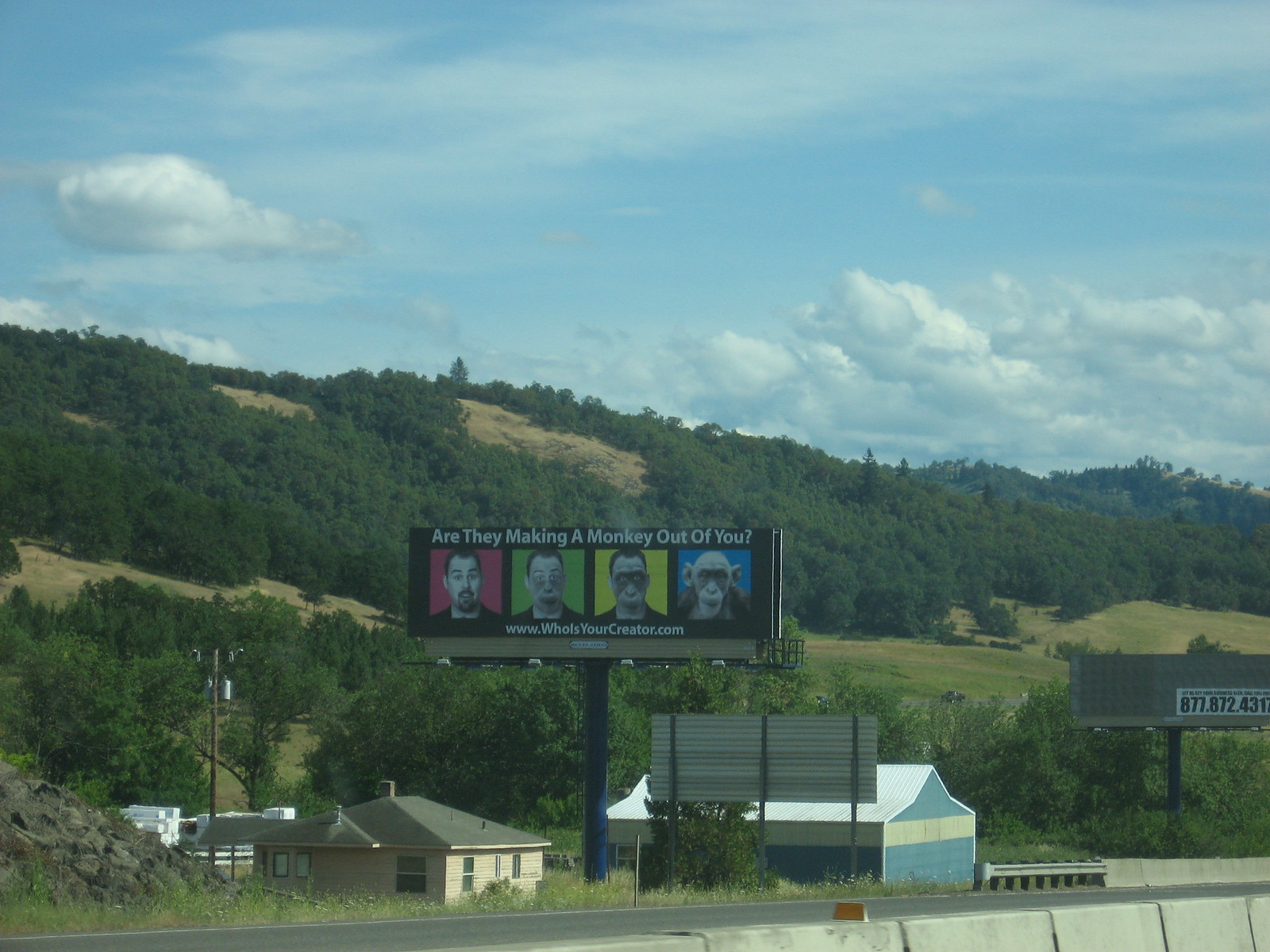The image is a slightly wider-than-tall outdoor scene featuring a partly cloudy sky at the top. Roughly a third of the way down is a lush, green hillside covered mostly with tall trees, interspersed with gaps of grass. This hill extends downward to about 80% of the image, leading to the foreground, where several buildings and houses are situated. Among these structures, there is a light blue barn centrally located, a tan house to the left, and a few more house roofs visible on the left side. 

Prominently placed slightly left of center is a tall billboard. The billboard displays the text "Are they making a monkey out of you?" and features four panels depicting a man gradually transforming into a monkey, promoting the website www.whosyourcreator.com. Below the billboard and in the foreground, there is an interstate road lined with a short white wall, adding to the suburban setting. The sky, with its mix of white billowy clouds and patches of blue, completes the detailed and dynamic scene.